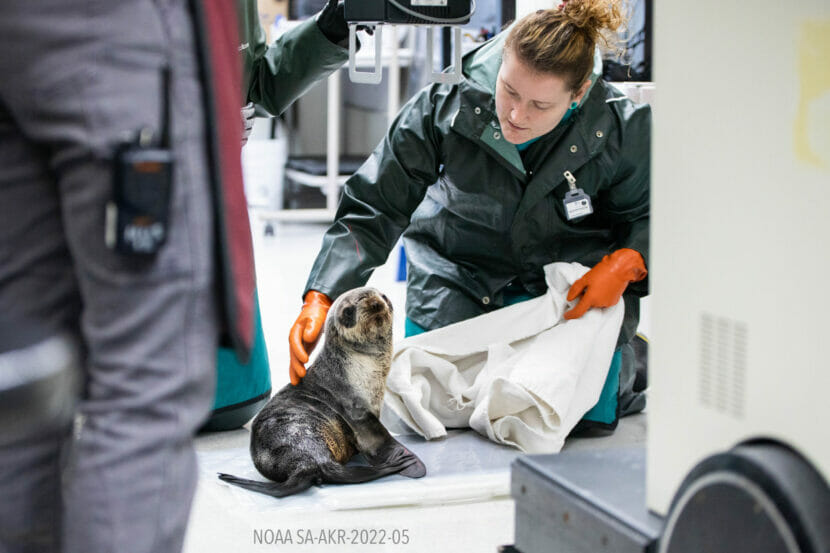In an indoor setting that appears to be an animal rescue center or clinic, a woman is seen caring for a baby seal. She is dressed in a dark green raincoat and orange rubber gloves, and her light brown hair is tied up in a ponytail or bun. With a focused expression, she gently touches the baby seal, which rests on a mat on the floor. The seal, which has a black back and a white underbelly, appears to be in need of medical attention. The woman holds towels, possibly preparing to clean the animal. A partially visible figure, identifiable by their gray pants and a walkie-talkie attached to their pocket, is seen standing nearby and interacting with equipment beside her. The letters "NOAASA-AKR-2022-05" are visible below the seal, marking its identification in the facility. The overall scene conveys a sense of care and urgency, highlighting the woman's efforts to aid the distressed seal.